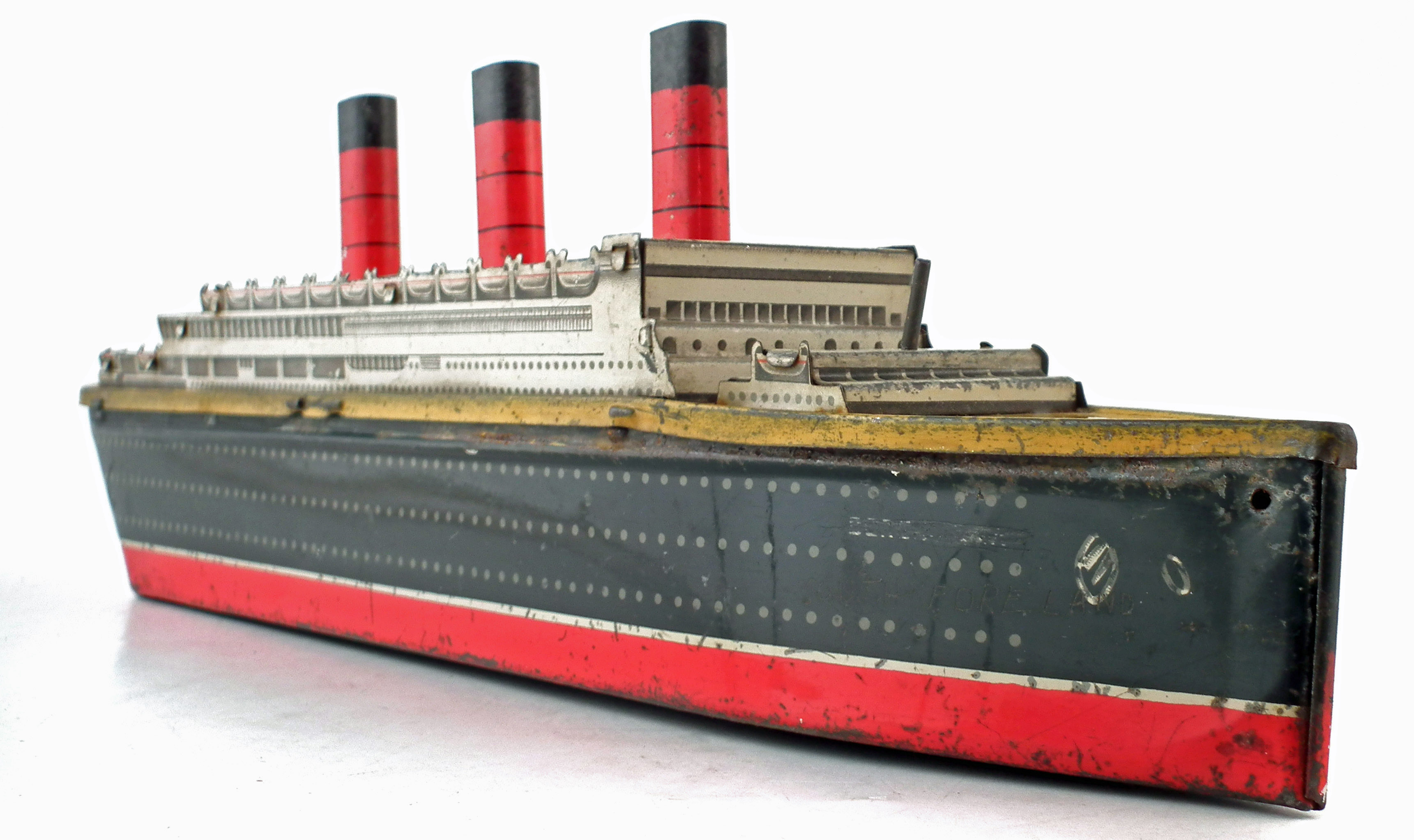Against a stark white background with subtle grey shadowing, an image features a detailed vintage model or illustration of a ship constructed from metal, perhaps aluminum or tin. The ship's upper section is a gleaming silver with a yellow trim running along its side, below which lies a black section adorned with three lines of small white dots. Beneath this, a slender silver-white band separates the top from the vivid red bottom hull, which shows signs of wear and tear. The vessel's deck area is marked with a yellow band, leading up to three prominent red smokestacks. Each smokestack has a red body segmented by two black lines, capped by a smooth black top. The ship’s front displays a small hole on the hull, likely intended for a rope. This intricately detailed model, evocative of historic liners like the Titanic, showcases an array of colors and textures that make it stand out sharply against the plain background.